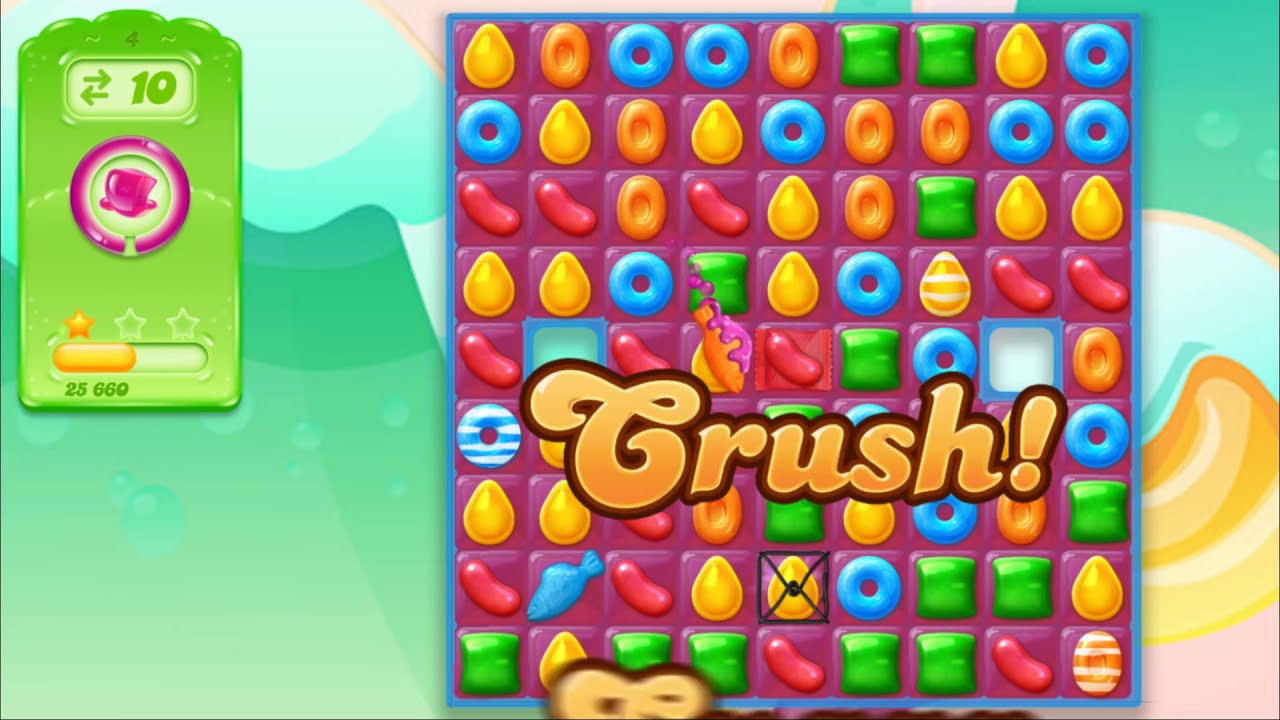The image is a detailed screenshot of the mobile game app, likely Candy Crush. Dominating the center is a checkerboard-like grid displaying 100 colorful candy pieces, including turquoise lemon drops, green mints, blue donuts, red jelly beans, and white squares. Overlapping this grid in bold, gradient orange letters is the word "Crush!" with an exclamation mark at the end. The background features abstract shapes in pastel shades of green, blue, and yellow, echoing the candy colors.

On the left side of the screen, there is a card-like element with a rectangular shape featuring a number 10, flanked by right and left pointing arrows. Below this card, there is a pink circle containing a top hat. Underneath, there are three star shapes; the leftmost star is filled in yellow and associates with the score of 25,660. Above these stars, a progress bar stretches horizontally. The right side mirrors the colorful aesthetic with more pastel hues. This immersive and vibrant layout strongly presents the visual identity of the game, capturing attention with its lively and engaging elements.